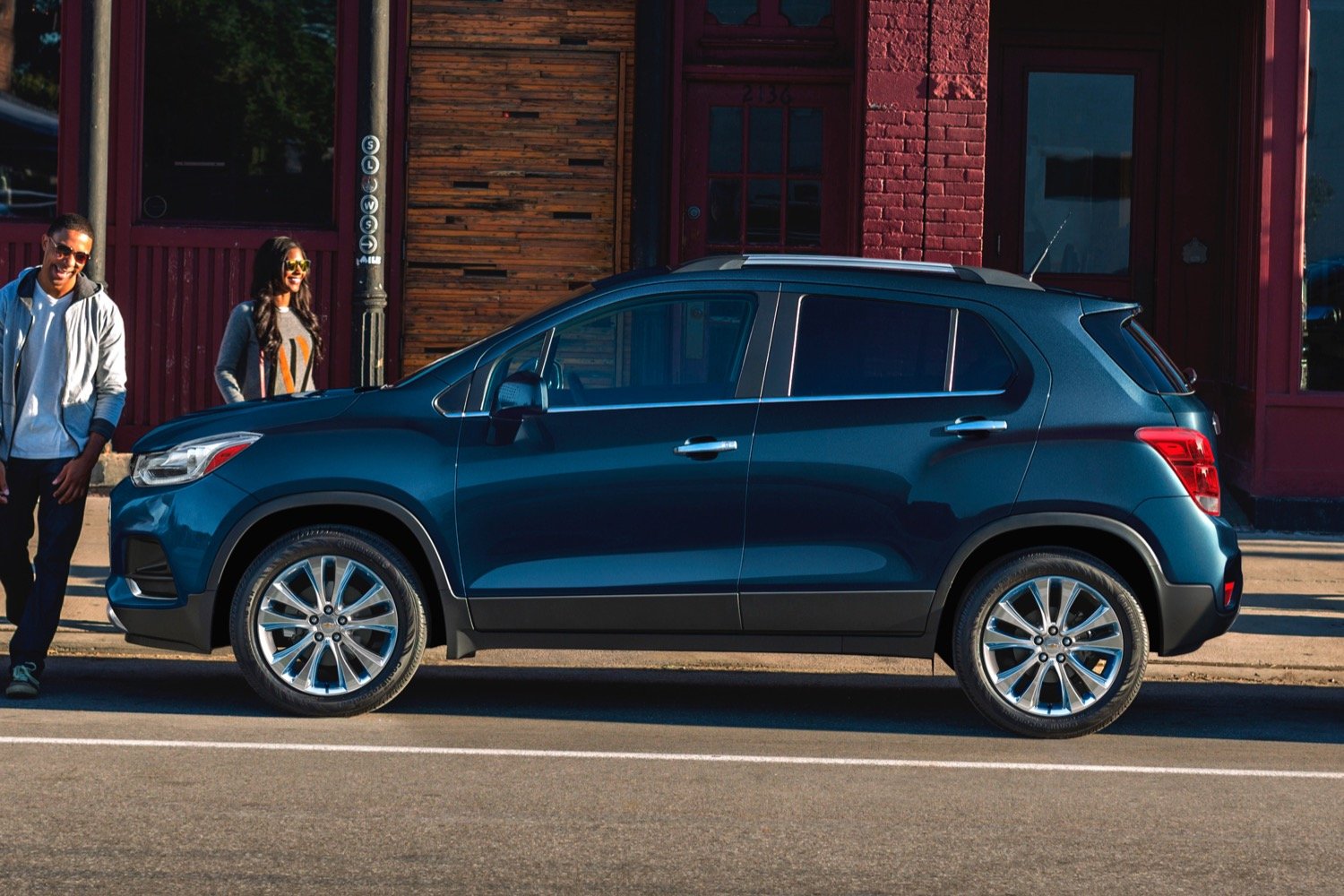In this modern urban scene, a sleek, dark blue SUV with a four-door configuration is prominently parked along a clean city street. The vehicle, facing towards the left, gleams under the soft light, which hints at either sunrise or sunset. The SUV sits parallel-parked next to a massive, old red-brick building with gigantic doors and large windows, blending seamlessly with the city's historical architecture. The street showcases a palette of reds, browns, blacks, and beiges, contributing to the scene's cozy yet vibrant aesthetic.

Two casually dressed individuals, both smiling and sporting black sunglasses, add life to the photograph. They are both Black; the man on the left side of the image, wearing a white hoodie and black pants, appears to be crossing the street towards the driver’s side. The woman on the sidewalk, adorned in a gray sweater and sporting straight hair, seems to be heading towards the passenger side. Their relaxed and cheerful demeanor suggests a leisurely outing as they approach their modern SUV, ready to embark on their next adventure amidst the urban backdrop.